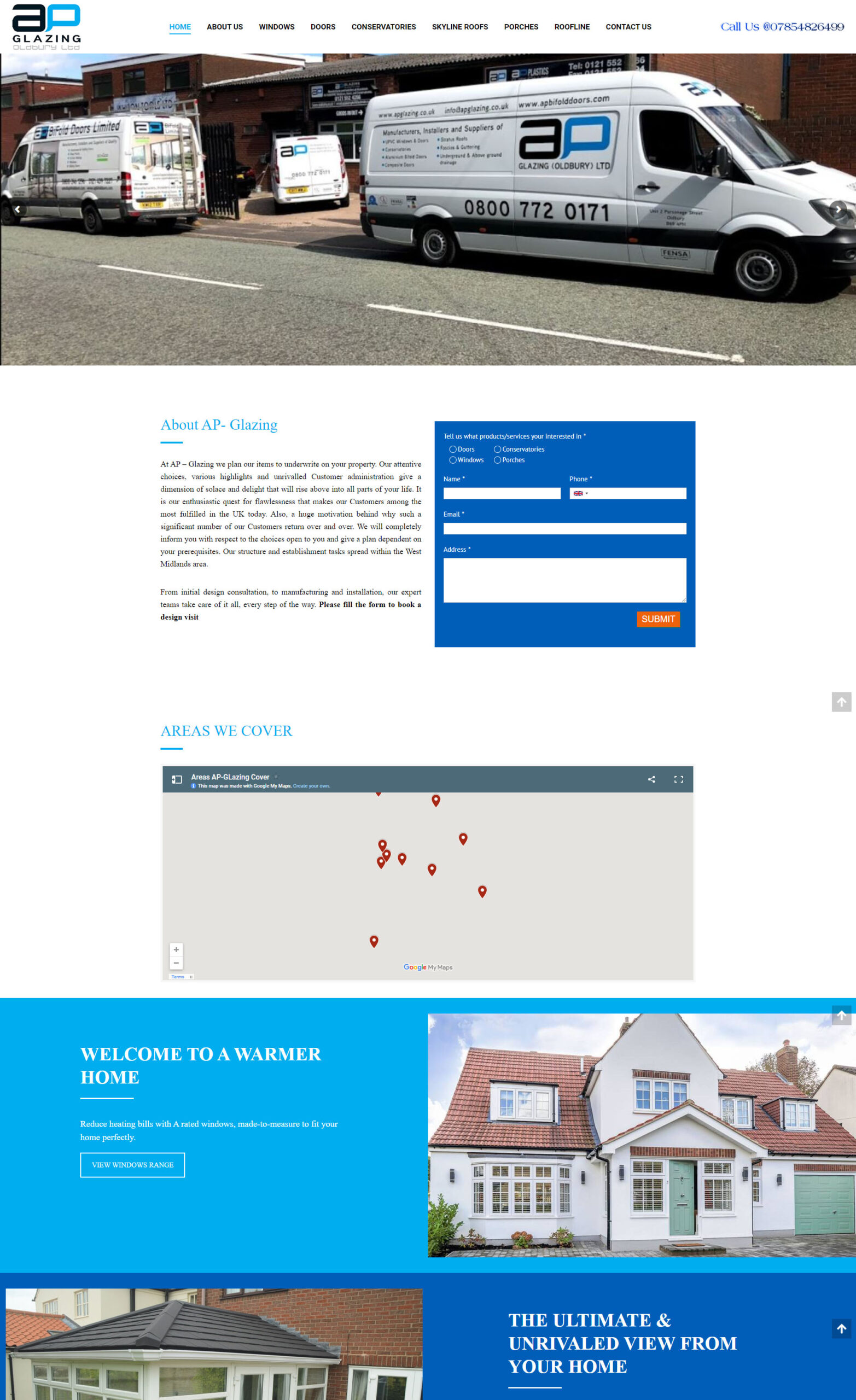Caption:

At the top of the image, a road is depicted with several white vans parked along the sidewalk, likely representing a fleet of service vehicles. In the upper left corner of the image, the lowercase letters "a" in black and "p" in blue, styled in block letters, are prominently featured. Below this, the word "GLAZING" is displayed in capital letters, suggesting that the service involves some form of glazing or home improvement. 

Adjacent to this, there's a labeled map area inside a gray square with several red dots, and the text "areas we cover" in blue above it, indicating the geographic regions serviced by the company. Further to the left, a blue square contains the white text "welcome to a warmer home." To the right of this text, there's an illustration of a house, characterized by its white exterior, brick red roof, and tall, elongated windows.

Beneath these elements, the phrase "The ultimate and unrivaled view from your home" is displayed, enhancing the impression of quality service that improves home aesthetics and comfort.